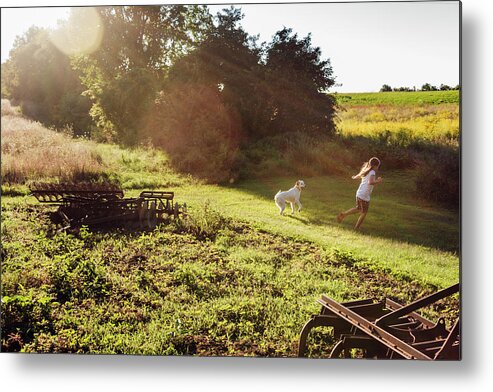This photograph captures a lively scene on a farm, framed by a thin black border and illuminated by bright sunlight streaming from the upper left corner. The sky stretches across the background in a dim, light grayish-blue hue, casting a serene atmosphere on the expansive, green landscape with various shades of lush grass. In the forefront, the rustic charm of old, metal farm equipment, possibly a broken plow, rests on the slightly rough grass.

Dominating the scene, a young girl dressed in a white outfit with a light brown ponytail sprints energetically through the field, her leg mid-air in motion. To her left, a medium-sized white dog playfully chases her, its legs lifted joyously. They are both running down a gentle hillside, adding a dynamic sense of movement to the idyllic countryside. Behind them, thick clusters of dark green bushes and possibly a large tree sit under the bright, shadow-casting sunlight, while the expansive fields stretch out in the distance under the soft, light grayish-blue sky.